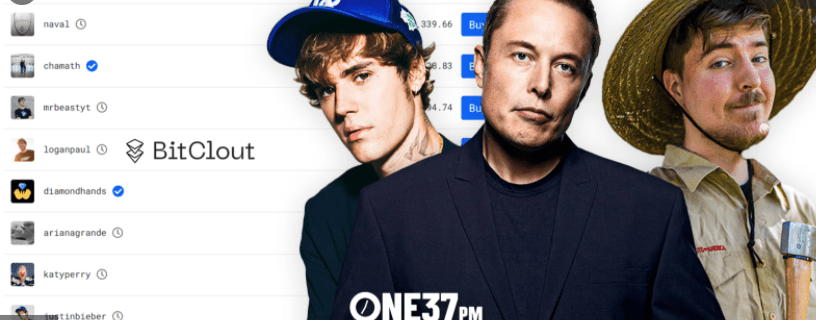The screenshot captures a segment of a website interface, notably devoid of any browser frame or URL bar, providing a seamless view of the content. The layout is divided into two primary sections. 

On the left-hand side, there is a vertical list featuring a series of icons. The icons are blurred but appear predominantly to be headshots of various individuals. Adjacent to these icons, written in gray text, are the names "Naval, Chamath, MrBeastYT, Logan Paul, Diamond Hands, Ariana Grande, Katy Perry, and Justin Bieber." Notably, "Chamath" and "Diamond Hands" are marked with blue checkmarks, indicating verified accounts, whereas the majority of the others are accompanied by gray clocks instead.

The right-hand section, centered on a white background, displays the title "Bit Cloud" in gray text. Adjacent to this, on the far right, there is an image depicting three men. Justin Bieber is positioned on the left, with Elon Musk standing directly in front of him. To the right stands a man whose identity is unclear; he is distinguished by a tan straw hat, a khaki-colored shirt, and what appears to be an axe in his hand. At the lower left part of Elon Musk's shirt, the text "1.37 p.m." is prominently displayed in bold white letters.